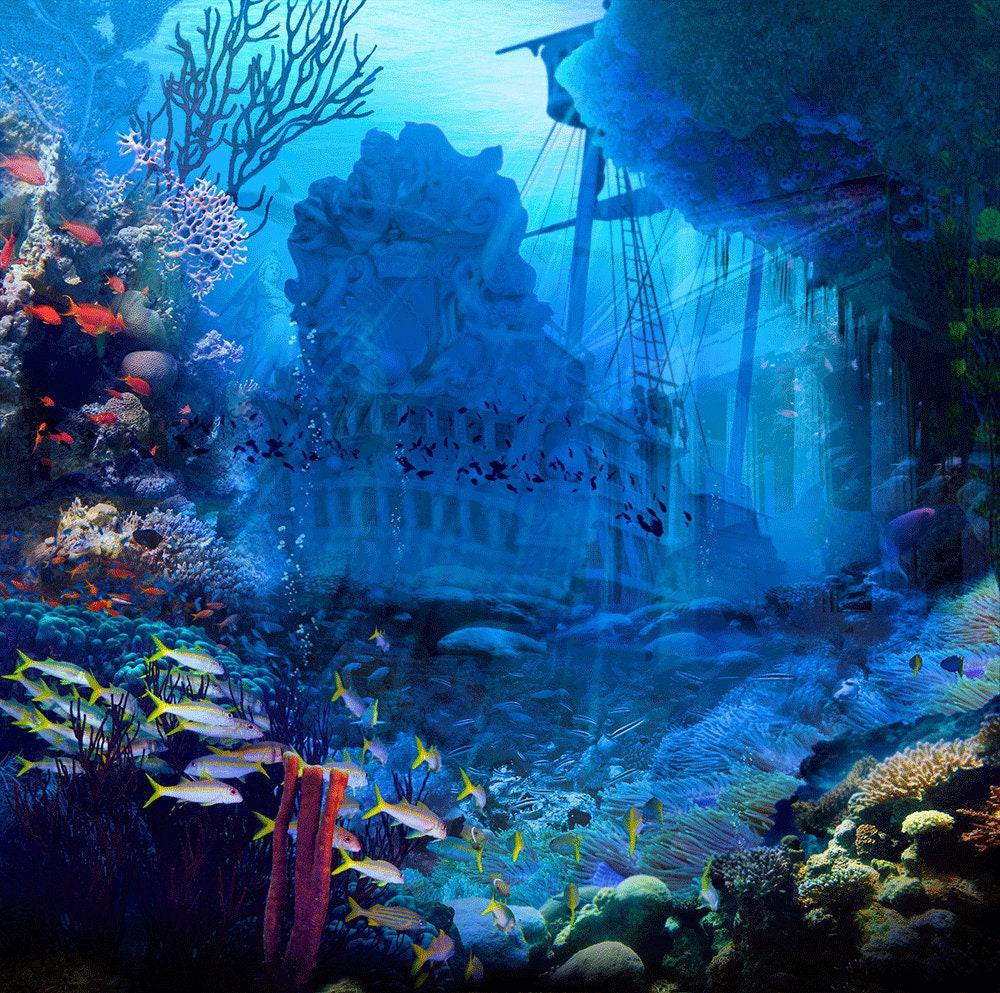This image appears to be a detailed painting of an underwater shipwreck scene. At the center of the composition, an old pirate ship rests on the ocean floor, its original colors obscured by age and aquatic growth. The ship features two rows of windows and a large, face-like statue at its bow, with a wooden mast behind it, adorned with cables.

The background is awash with the deep blue hues of ocean water, while the foreground bursts with life and color. Numerous fish populate the scene, particularly along the left and bottom edges. The fish on the left are predominantly orange, while those at the bottom exhibit silver bodies with yellow tails. Surrounding the shipwreck, vibrant coral formations in shades of white, blue, and other colors thrive, along with an assortment of plant life and rocks.

A bit of rock formation is visible in the top right corner, suggesting an underwater cliff or cave area. The bottom right corner is well-lit, teeming with various colored corals and rocks. This intricate and vibrant depiction of an underwater world captures the mystery and beauty of a long-lost pirate ship amid a thriving aquatic ecosystem.